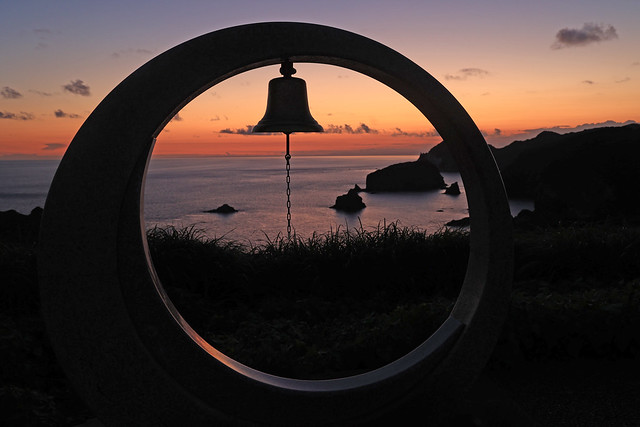The photo captures a serene outdoor scene at sunset, showcasing a picturesque blend of natural and man-made elements. In the foreground, a large, hollow circular structure dominates the composition. Suspended from the top of this frame is a bell, reminiscent of the Liberty Bell, with a chain hanging down its center, giving the impression of a bell ringer. The bell and chain appear as silhouettes due to the low light conditions.

Through the circular frame, the viewer is treated to a stunning view of a large body of water, possibly an inlet or bay, leading out to the horizon where the sun is just setting. The sky is beautifully gradient, transitioning from a deep reddish hue near the horizon, through bands of yellow and orange, to a dark blue and purple at the top. Although the sky is mostly clear, there are scattered clouds adding texture to the scene.

In the midground, large rock formations and grassy areas fringe the water, adding depth and contrast to the image. The rocks are dark and shadowy, blending seamlessly with the silhouette of the bell and the circular frame, while the grass offers a softer texture. The overall scene is tranquil and evocative, capturing the peacefulness of the closing day.